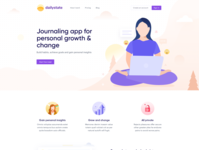This screenshot is quite small and blurry, making it difficult to discern details. At the top, on the left side, the website name is visible, followed by an unreadable menu list consisting of three options. On the right side, there's a noticeable purple button. The right section of the image features a cartoonish illustration depicting a woman in a lotus pose with a laptop on her lap. She has black hair, a blank face without features, and is dressed in a short-sleeved purple shirt and purple pants, sitting with bare feet. The background is adorned with a light purple design including some trees.

To the left of the illustration, the text reads "Journaling app for personal growth and change," with another purple button located beneath this text. Below this section, set against a white background, are three circular images, each accompanied by a heading and a short description. However, due to the image's blurriness, these details are indistinguishable. Some additional text appears to be cut off by the limits of the screenshot.